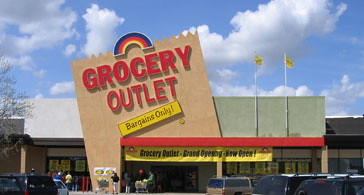This rectangular photograph captures a vibrant scene of a grocery store from the parking lot. Dominating the image is a large brown angled sign resembling a billboard, prominently displaying "Grocery Outlet" beneath a rainbow featuring blue, red, and yellow stripes. Below this, a bold red banner reads "Bargains Only."

Further down, there is a long yellow sign indicating "Grocery Outlet Grand Opening Now Open" written in black text. This sign spans the storefront, which also features a row of approximately ten windows, each with a yellow sun graphic suggesting discounts and promotions.

The foreground includes a bright, reflective view of the parking lot, showcasing several cars and shoppers, some of whom are pushing grocery carts. A greeter waves at people entering or exiting the store. Two metal poles on the right side of the roof fly yellow flags, adding to the celebratory atmosphere.

Above, the sky is a brilliant blue strewn with white, fluffy clouds, completing this lively and bustling scene of the grand opening event.